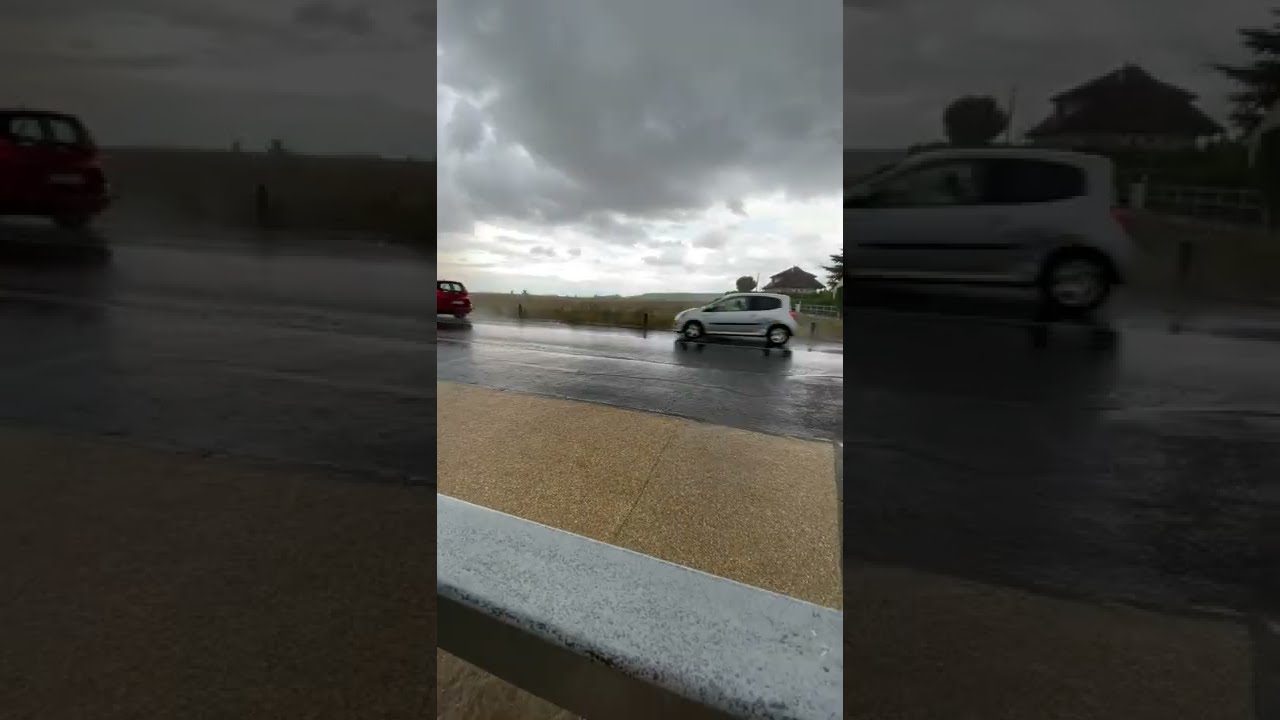On a rainy day, the image captures a road slick with moisture, under an ominous, dark gray sky filled with storm clouds. The scene is devoid of people, focusing instead on two cars traveling along the wet highway. To the right, there is a silver two-door hatchback, and to its left, a red car with a white license plate. A sand-brown walkway with a gray curb appears in the foreground, indicating a separation from the road. Across from the road, a tan colored field filled with grass stretches out, with a house featuring a brown roof and gray walls visible in the far distance on the right. No cyclists or pedestrians are seen, underscoring the solitary and wet atmosphere of the moment.